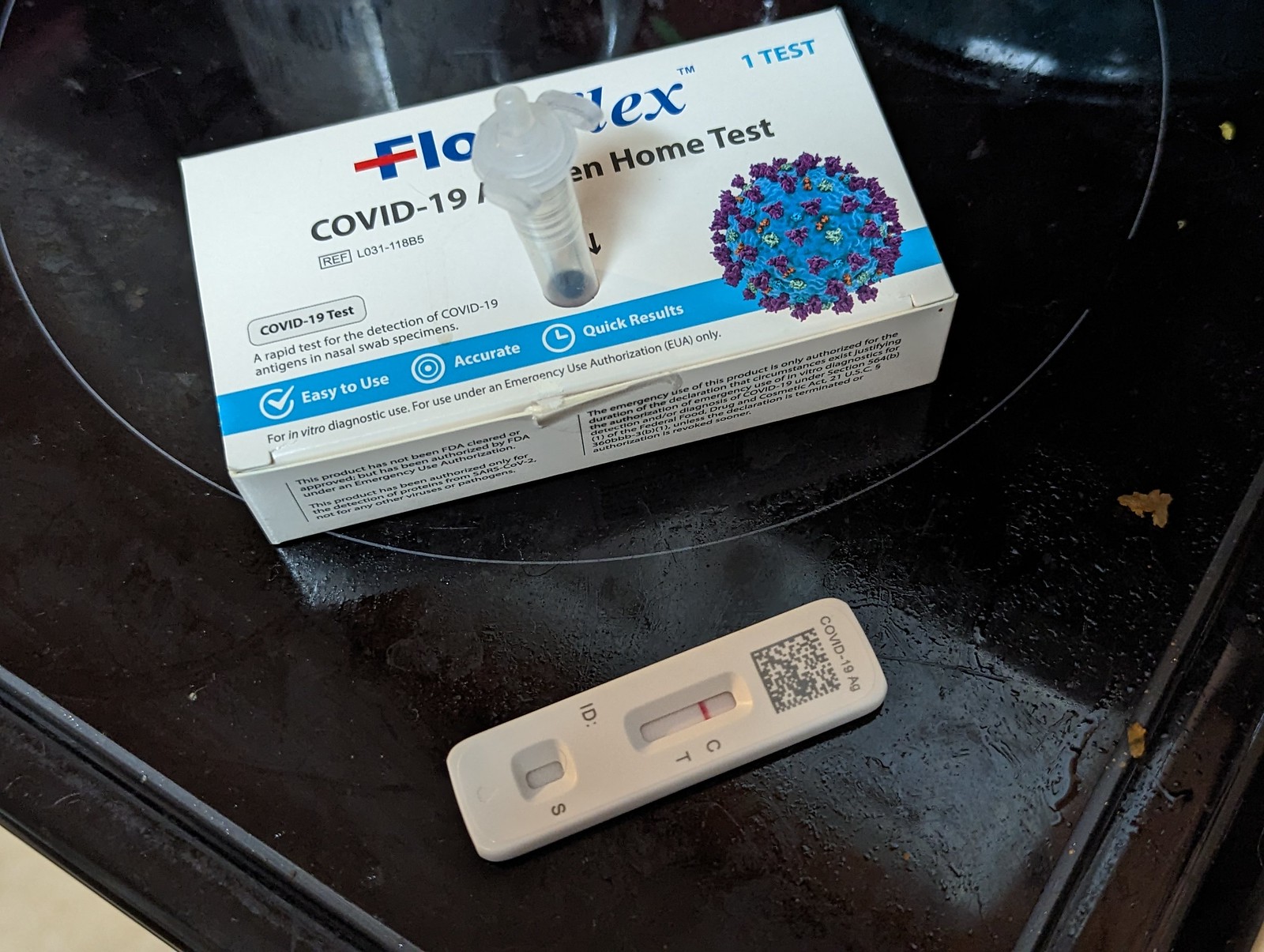The photo depicts a white cardboard box positioned on a greasy, flat cooktop stove, indicating frequent use for frying foods. The box features blue lettering and is partially obscured by a small, tubular plastic device with a cap. The visible text reads "Flow Something EX™" and "One Test," along with "COVID-19" followed by an obscured section and "Home Test," suggesting it is a COVID-19 at-home test kit. Also on the stove is a white plastic rectangular piece with a small window, showing a red line next to the letter 'C' but no line next to the letter 'T.'